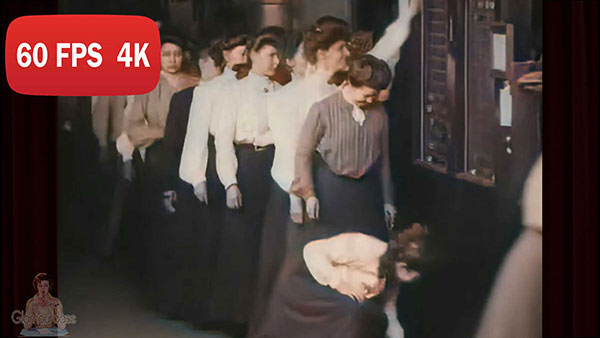The image appears to be a screen grab from a movie, depicting an old photograph of women, likely in their 20s to 40s, standing in a line, seemingly waiting to punch in at work. These women are dressed in conservative attire, featuring buttoned-up blouses in varying colors—white, brown, and pink—with lace and frills. They all have dark hair styled in neat updos and are wearing long, matching gray skirts. At the front of the line, one woman is bending down to pick up what appears to be her dropped punch card. The woman directly behind her observes with a smile, finding the situation amusing, while she reaches up to retrieve her own punch card. The rest of the women in line are waiting patiently, dressed similarly in long skirts and buttoned blouses. In the top left corner of the image, there is a red rectangle with white text that reads "60fps 4K," indicating a high-quality digital capture. The background suggests the setting is outside a time clock, preparing for a day at work.